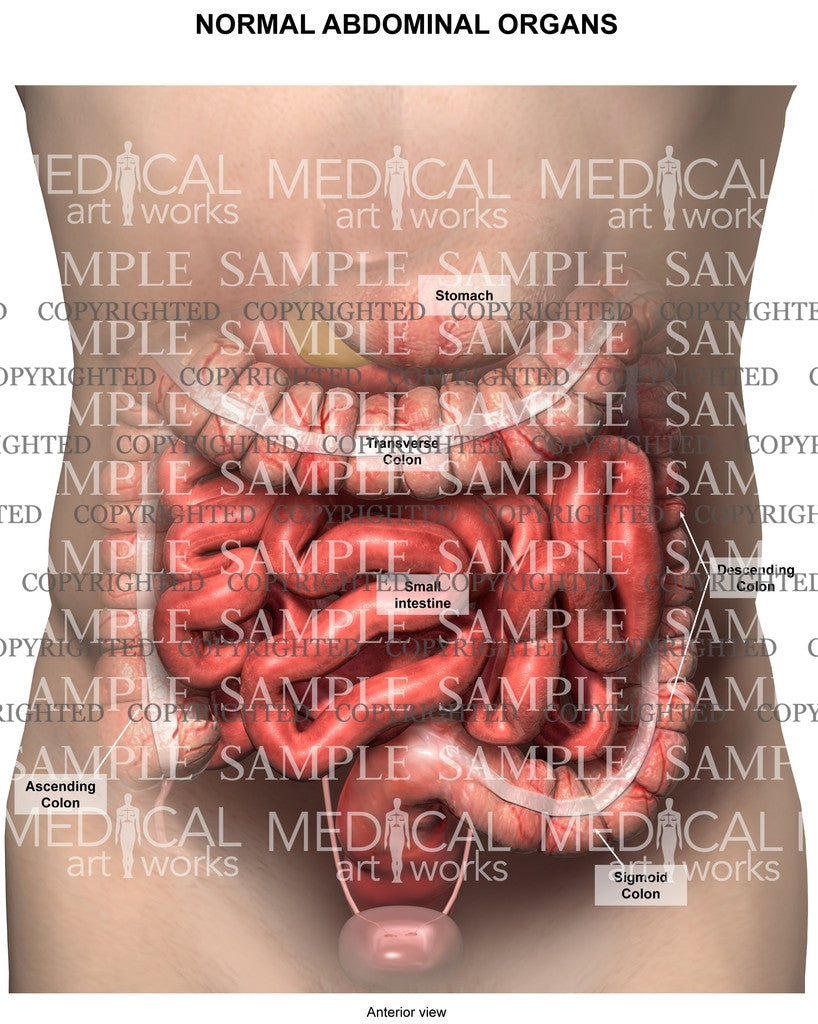An artistic medical illustration depicts the detailed anatomical structure of the human large and small intestines within the midsection of a Caucasian person's torso. The illustration resembles an x-ray view, revealing the internal positioning of various organs. Key parts are labeled, including the stomach, transverse colon, small intestine, descending colon, sigmoid colon, and ascending colon. The top of the image is marked with the title "Normal Abdominal Organs." Throughout the image, the words "medical artworks" are prominently displayed alongside a diagram of a person. A watermark reading "copyrighted" and "sample" covers the entire picture. At the bottom, in small black letters, the image is further labeled as an "interior view." The detailed and professional quality of the illustration suggests it is suited for use in a medical textbook.